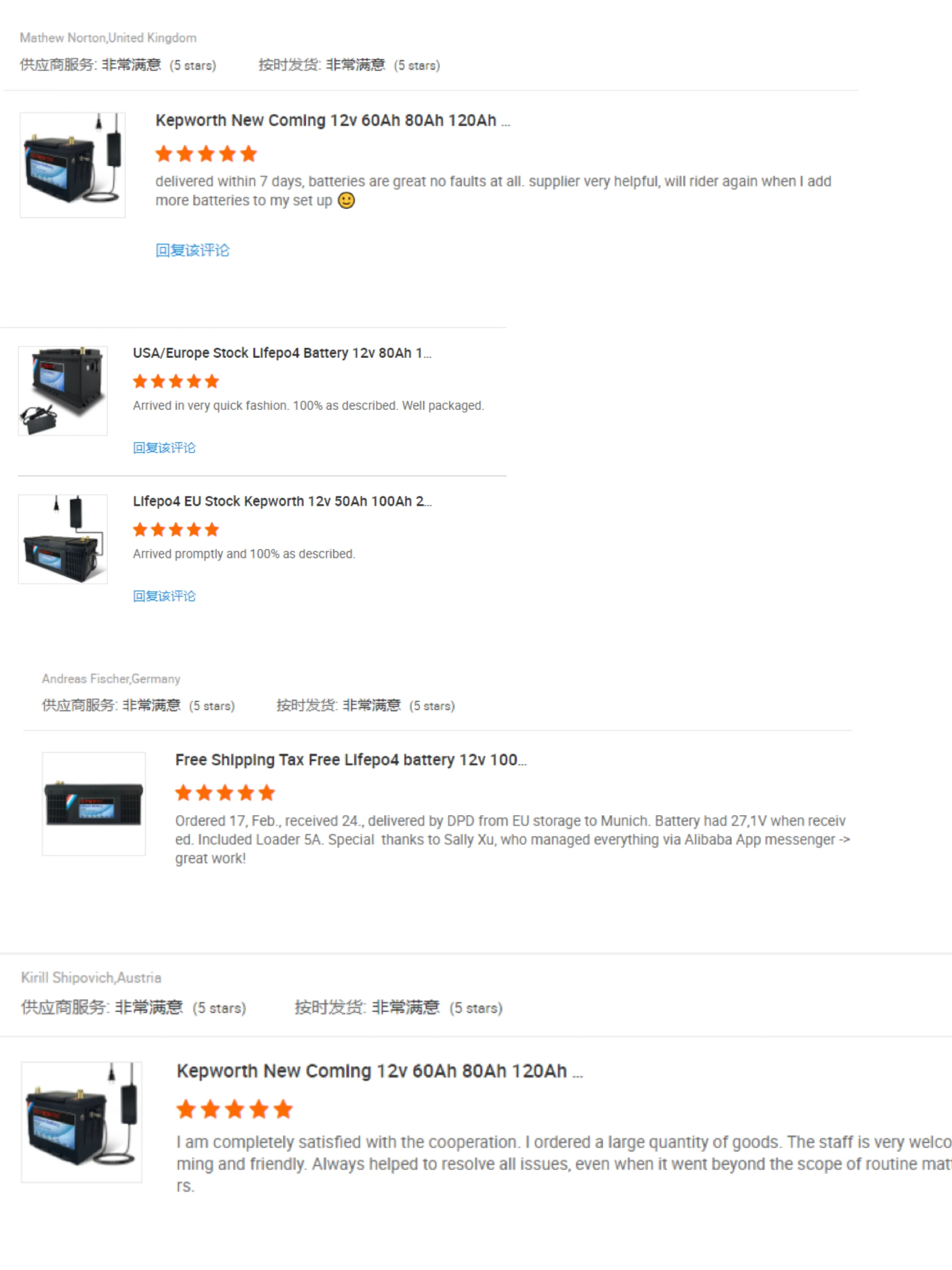A pristine white background showcases a variety of high-quality battery products. Featured prominently are Kepworth's new arrivals: 12V60Ah, 12V80Ah, and 12V120Ah batteries, each highly rated with five stars. Alongside these are USA and Europe stock LiFePO4 batteries, including a 12V88Ah model and a 12V100Ah version, both also boasting five-star ratings. These batteries offer free and tax-free shipping, making them an attractive option for customers. The user experience is enhanced by the exceptional customer service, with friendly and welcoming staff that have left me completely satisfied with my large purchase.